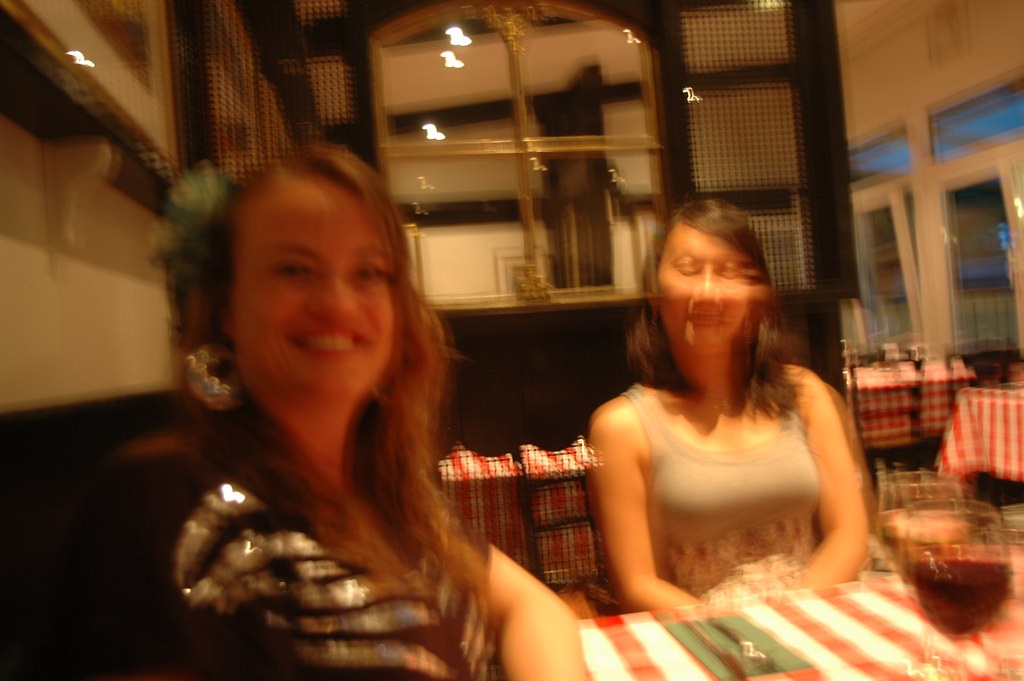Two young women are enjoying a meal at a quaint, moderately upscale restaurant. They are seated side by side at a table that appears to be part of a booth setup, with the woman on the left leaning against a wall that features a window, providing a view into another section of the dining area. The restaurant exudes a cozy atmosphere, accentuated by three visible tables, each adorned with classic red and white checkered tablecloths. The woman on the left is dressed in a shiny silver striped top and matching silver earrings that catch the light, adding a touch of elegance to her look. Beside her, the other woman, with her long brown hair flowing over her shoulders, is wearing a casual tank top. They are both seated comfortably at the table, seemingly immersed in conversation or enjoying the ambiance as someone, possibly seated next to the woman on the left, captures this candid moment.